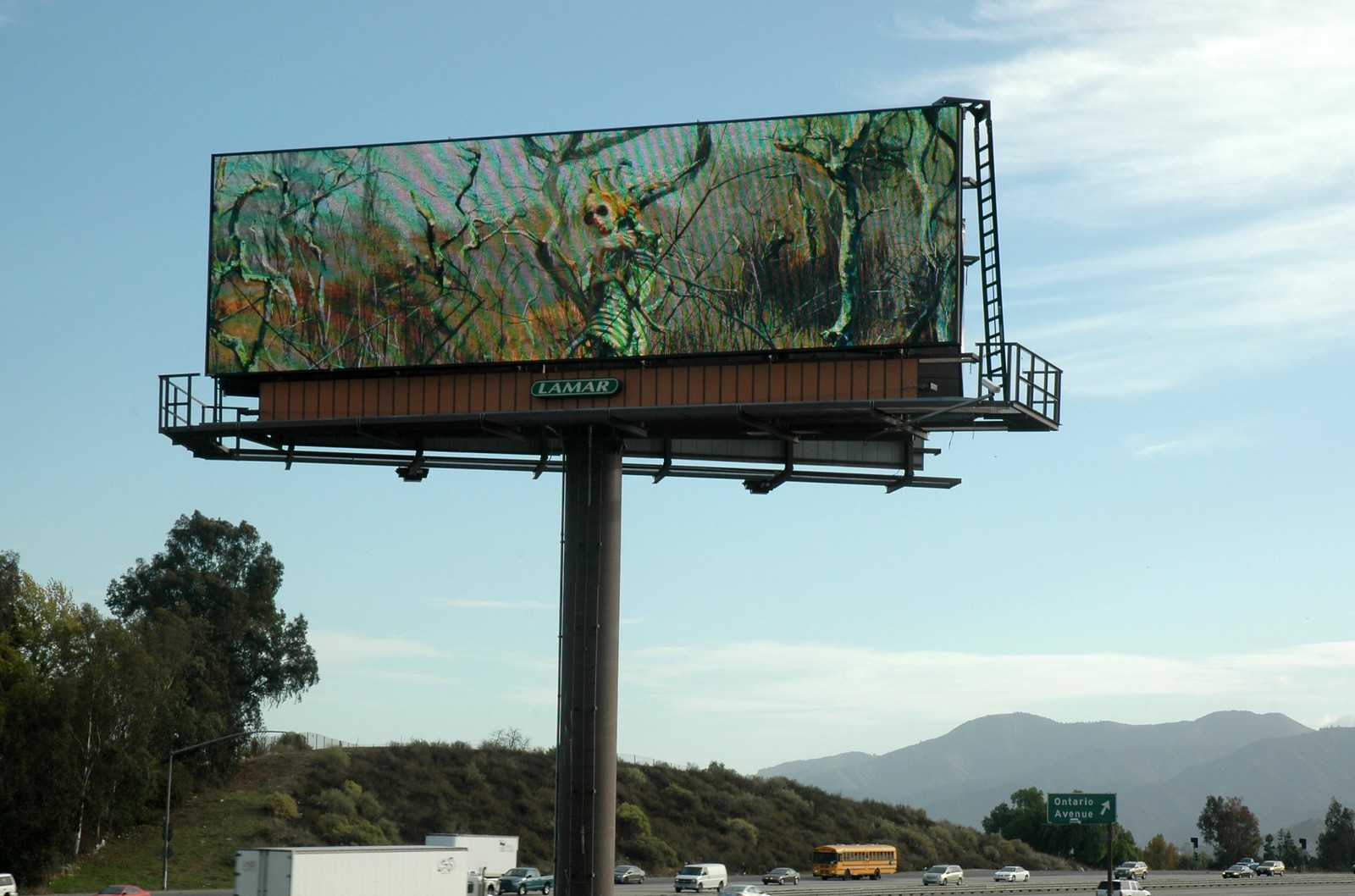The image showcases a tall, cylindrical black metal pole supporting a large rectangular billboard high in the sky, with a grey ladder attached to its side for access. The billboard stands prominently against a blue sky interspersed with wispy clouds, and distant silhouettes of mountains can be seen. The sign features a spooky scene with leafless trees, some appearing to have wings, adding to the eerie ambiance. A central figure with blonde hair, black sunglasses, and small horns, possibly part of a costume, is depicted, surrounded by dark, vine-like elements and a mostly brown and blue background, suggesting a forested area. Below the graphic, a black box with "Lamar" written inside sits at the bottom edge of the billboard. Nearby, there is a green street sign with white text that reads "Ontario Avenue," mounted on a black pole with a white arrow pointing upwards to the right. Below the elevated billboard, a bustling road is visible, populated with tiny vehicles such as a yellow school bus, cars, vans, and some semi-trucks, all surrounded by patches of green trees and bushes. There is another billboard in the background, facing away from this one.